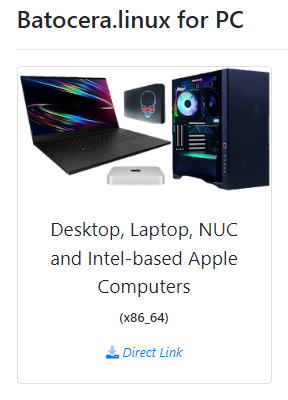This image is an advertisement, likely featured on a website for shopping. It has a clean, minimalistic design with either a black or white background. At the top, in bold black text, the ad reads "batocera.linux for PC." Below this, there is a thin gray line followed by a thin gray box outline, creating a focal point for the main visual elements.

Inside the gray box, the ad showcases an open black laptop displaying a vibrant rainbow screensaver. Adjacent to the laptop is a black desktop computer tower, illuminated from within by mesmerizing rainbow-colored LED lights, including a striking rainbow LED fan. Also within the box are two computer components: one is black with a visually intense skull featuring glowing red eyes, and the other is a sleek white component.

Further down in bold black text, the ad lists, "desktop, laptop, NUC and Intel-based Apple computers," broadly indicating the range of compatible devices. At the bottom of the advertisement, a prominent blue hyperlink invites users to take direct action.